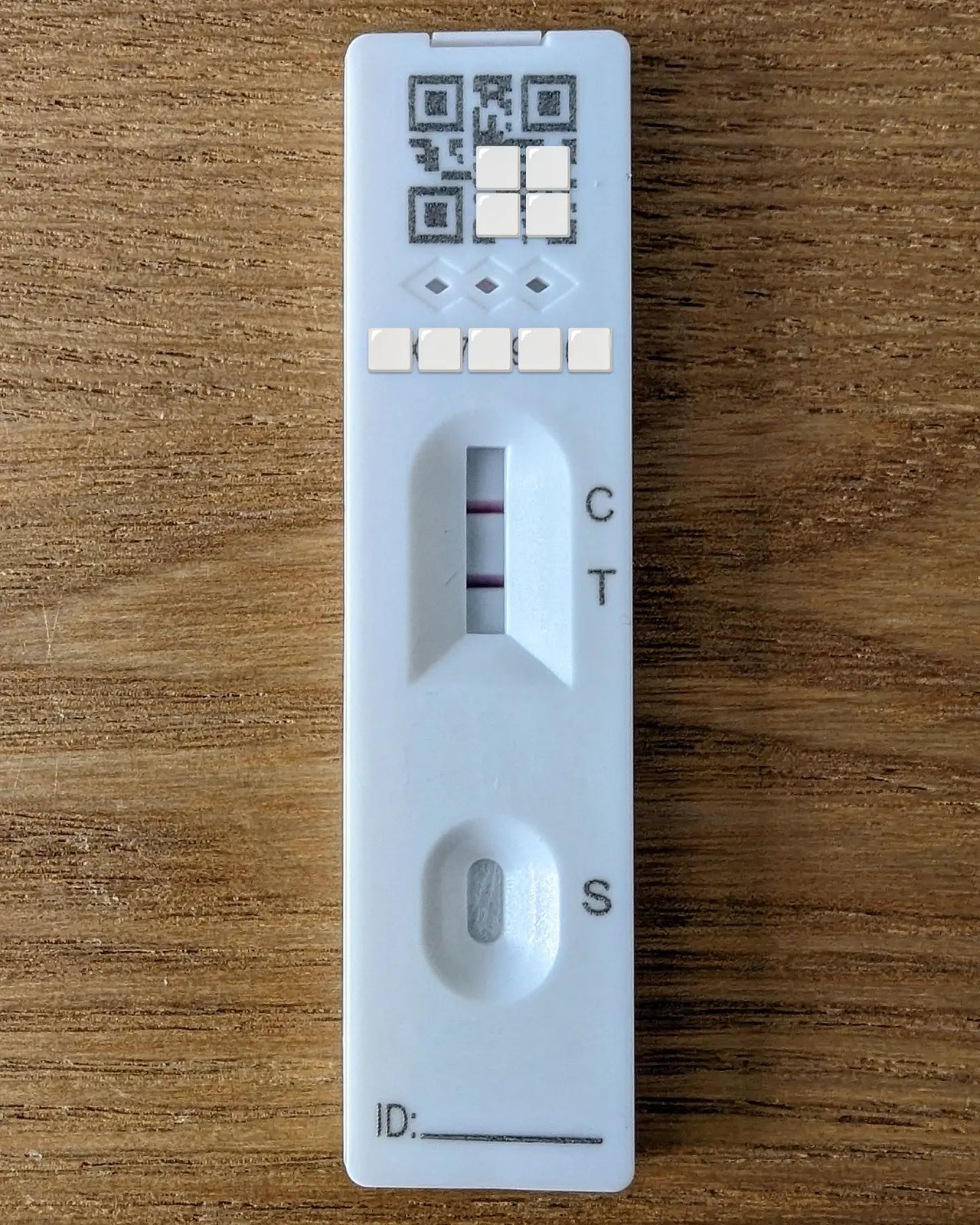An overhead photograph captures a wooden table with a baby blue rectangular object placed prominently. The object, significantly taller than it is wide, could potentially be a COVID test kit. 

At the top center of the object, there is a black QR code occupying approximately 25% of the space, with four white squares situated in the bottom right corner of the QR code. Beneath this QR code, there are three intersecting diamond shapes, each intersected at their vertices, creating a complex pattern. Within the larger intersecting diamonds are three smaller, non-intersecting diamond shapes.

Below the diamond patterns, there are five white squares aligned horizontally side by side. Beneath these squares, a large horizontal rectangle is centrally positioned and divided vertically into three equal sections by two purplish-reddish lines. Adjacent to the top and bottom red lines on the right side, the letters "C" and "T" are marked, respectively.

Further down, the object features a vertically oriented rectangle with rounded top and bottom edges. To the right of this shape is the letter "S." At the very bottom of the object, the label "ID:" is followed by a lengthy black line, awaiting an intended inscription.